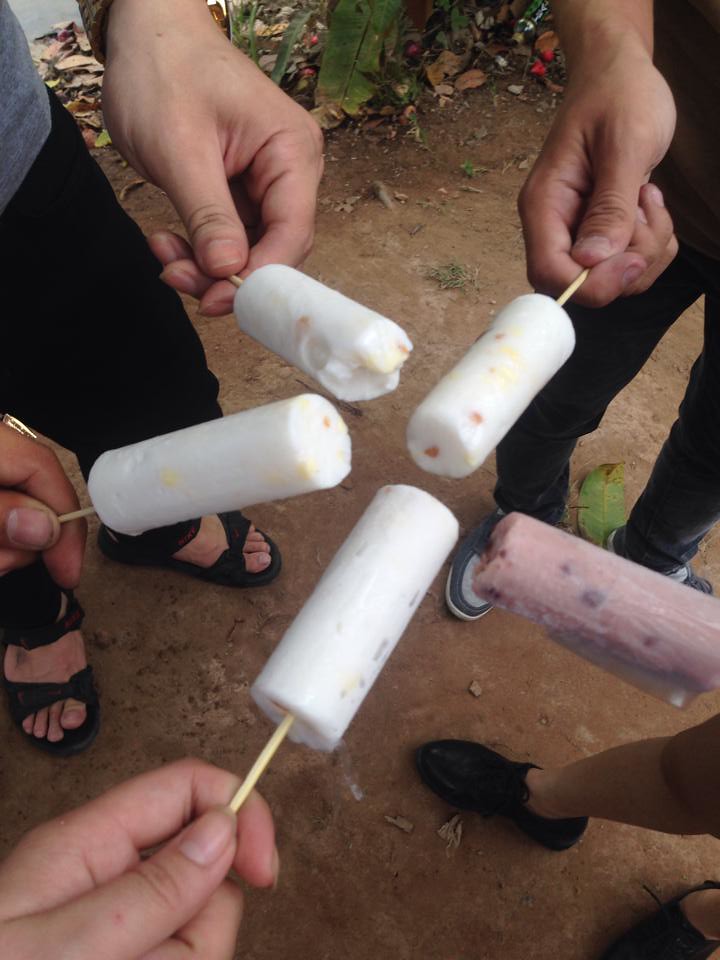The image depicts a sunny outdoor setting where five individuals are standing in a circle, each holding a popsicle towards the center, creating a star-like formation. The popsicles are cylindrical, resembling push pops but without the cardboard casing. Four of the popsicles are white with small brown and yellow specks, while the fifth popsicle, located at the bottom right, is a darker pinkish-purple color with black specks. The individuals holding the popsicles have lighter-toned skin, and we can see parts of their hands and feet in the image. The footwear visible includes black sneakers at the bottom right, black flip-flops at the middle left, and gray-white sneakers at the middle right. The individuals are standing on what appears to be dirt, suggesting they might be in a natural outdoor setting, possibly near woods or a casual outdoor area.